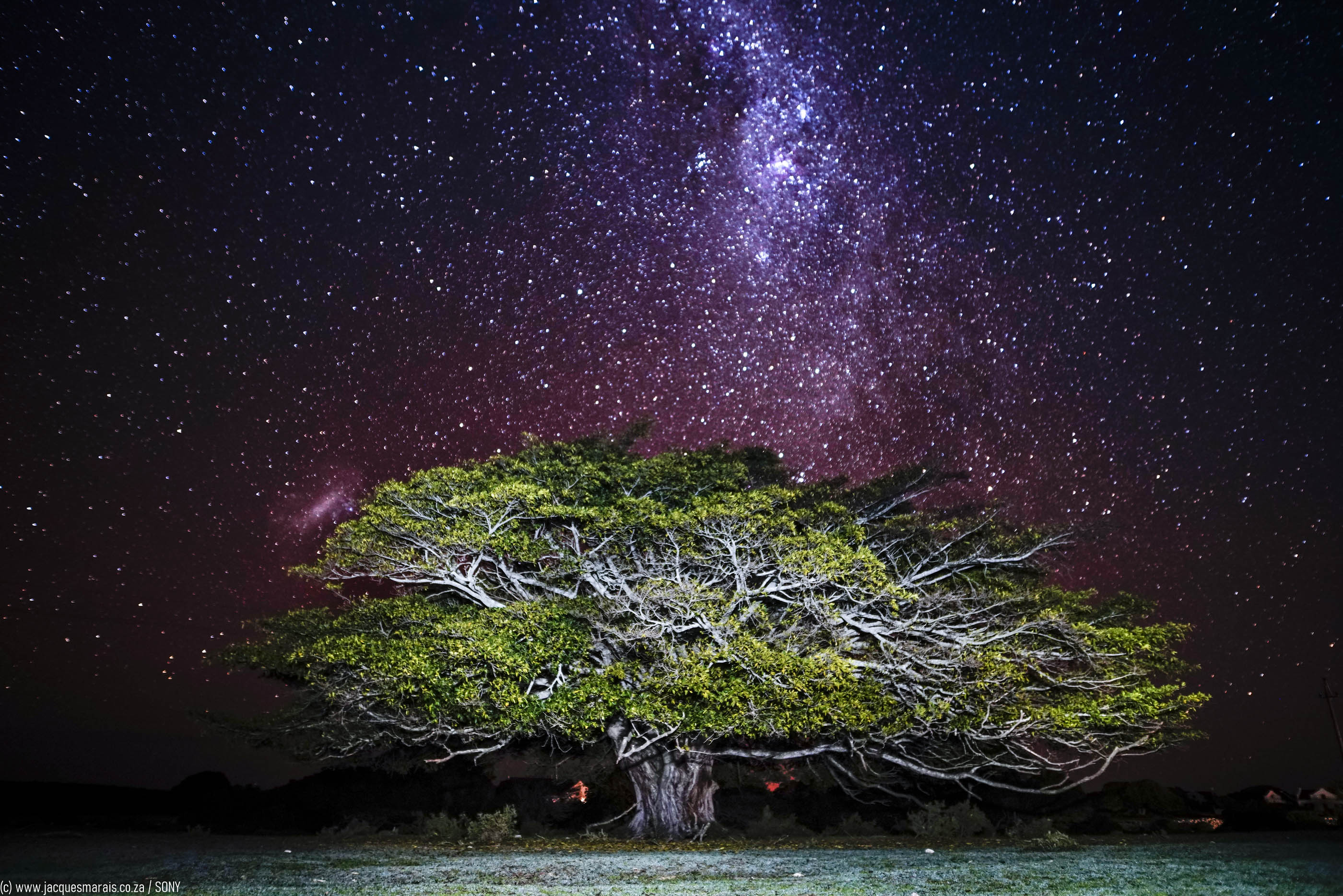In this stunning nighttime photograph, a massive, ancient deciduous tree dominates the foreground. Its wide trunk supports dramatically spread branches, which extend nearly twice the width of its height, creating a fan-like appearance of gnarly, almost white bark with patches of green foliage. Some branches appear bare or almost dead, adding to the tree's commanding yet eerie presence.

The sky above is clear, filled with countless bright stars clearly visible against the dark expanse. Among them, the Milky Way is prominently displayed, its nebula clouds adding a luminous, otherworldly glow to the scene. The ground around the tree features green grass, small shrubs, and scattered rocks, contributing to the tree's grounded, sturdy impression.

In the distance, faint red spots suggest either taillights or campfires, while off to the far right, there seem to be houses. This subtle lighting hints at a nearby road or settlement, adding depth to the scene. The whole photograph seems to capture a moment in time, possibly using a time-lapse to bring out the beautiful, star-filled sky and the detailed textures of this ancient tree. The overall composition combines natural grandeur with a touch of mystery, making it an absolutely stunning and detailed capture.